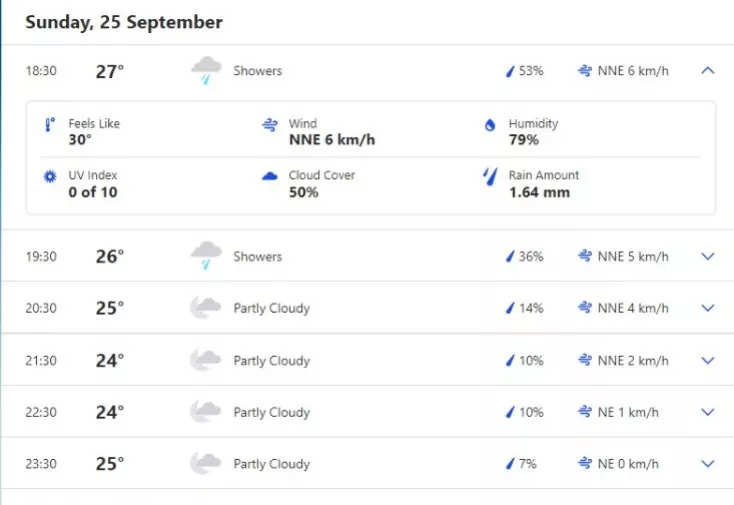On Sunday, 25th September 1830, the recorded weather conditions displayed a diverse range of meteorological data against a stark white background with detailed black text, some in bold to highlight temperatures. At 27 degrees Celsius, showers occurred with a 53% chance, blown by NNE winds at 6 kilometers per hour, making it feel like 30 degrees. Humidity stood at 79%, the UV index was 0 of 10, and cloud cover at 50% with rainfall totaling 1.64 millimeters.

By 19:30, the temperature slightly dipped to 26 degrees with a 36% chance of showers and NNE winds at 5 kilometers per hour. An hour later, at 20:30, the temperature relaxed into 25 degrees with partly cloudy skies and only a 14% chance of rain, accompanied by NNE winds at 4 kilometers per hour.

As the night continued, at 21:30, it was 24 degrees with partly cloudy conditions and a 10% chance of rain, NNE winds slowing to 2 kilometers per hour. By 22:30, the temperature and conditions remained consistent, with NNE winds further reducing to 1 kilometer per hour. Finally, at 23:30, the day concluded with 25 degrees, partly cloudy skies, a minimal 7% chance of rain, and calm NNE winds at 0 kilometers per hour.